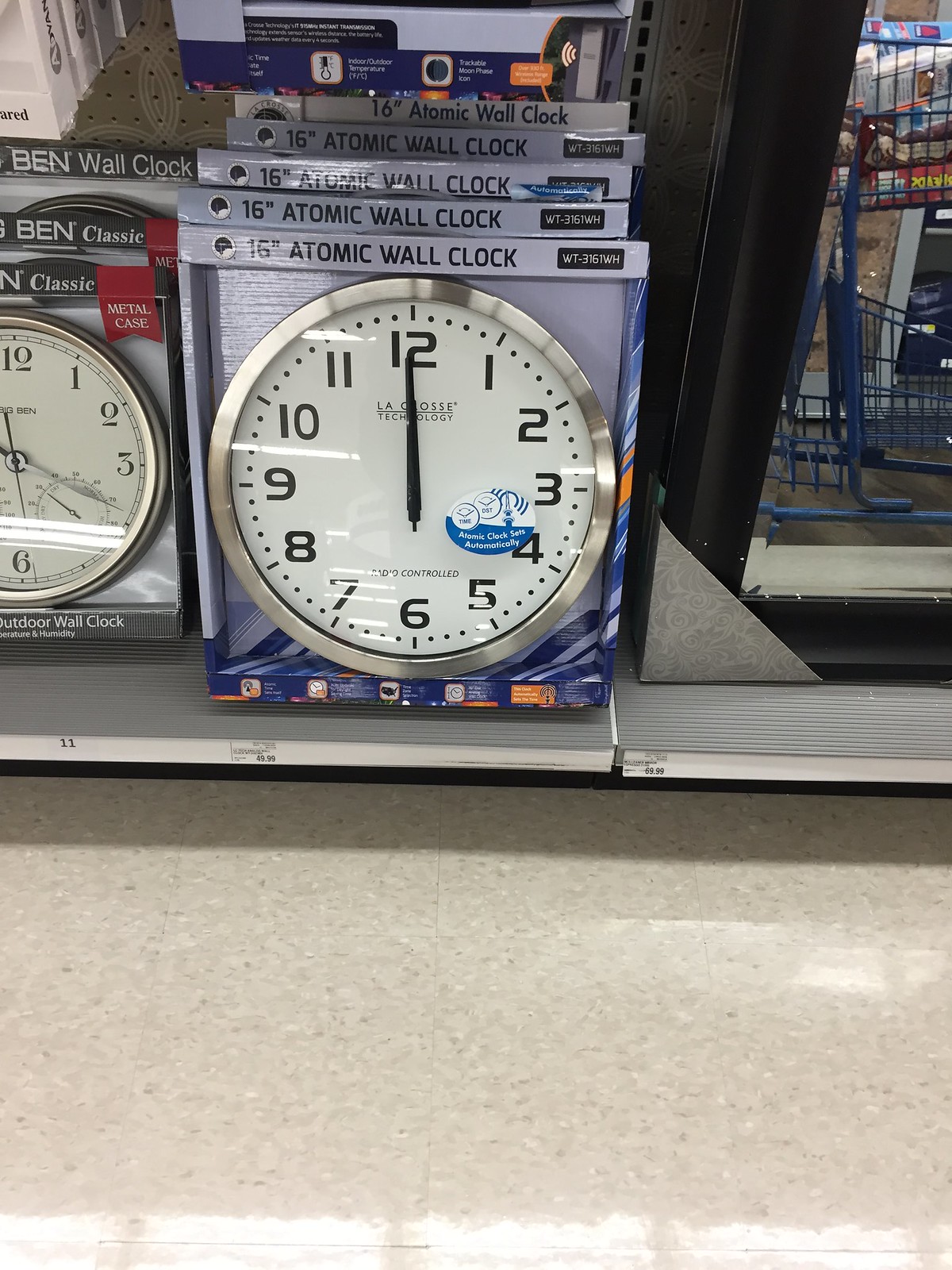This photograph, taken inside a retail store from a low vantage point near the ground, captures a clear view of the white tile flooring speckled with gray. The primary focus is a shelf displaying boxes of wall clocks for sale. Prominently featured is a square box labeled "16-Inch Atomic Wall Clock." The packaging is designed with a blue and white color scheme. The clock itself has a sleek, silver circular frame, with a straightforward design that includes numbered hours from twelve all the way around. The branded clock, which appears to be by Lacrosse or Lacoste, is highlighted by a blue and white sticker on the front of the box.